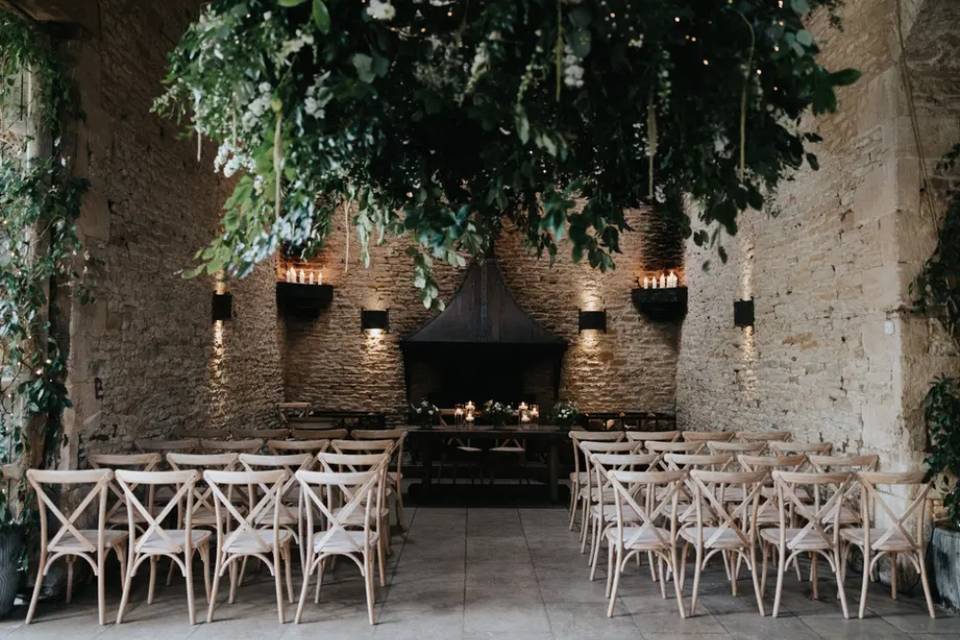This horizontal, rectangular image depicts an outdoor setup, likely for a wedding or special event. The scene is enclosed by off-white stone or brick walls that feature climbing vines with green leaves. Dominating the top of the image is a large tree with lush green foliage that creates a canopy effect, giving the space an intimate and shaded ambiance.

The flooring is made up of gray, concrete tiles with geometric patterns. The seating arrangement consists of white, four-legged wooden chairs with thin white cushions, arranged in rows of four on either side of a central aisle. These chairs have an X-cross back design and look somewhat basic in comfort.

At the focal point of the image is a raised platform at the end of the aisle, potentially the ceremony spot or a stage for performances. Around this platform, there are dark tables and a prominent black fireplace or structure that hangs from the ceiling. The area is decorated with accent lights, tables, and candles that add a soft, warm glow to the setting. Black shelves holding candles and black light fixtures emitting yellow light enhance the ambient mood of this picturesque setting.